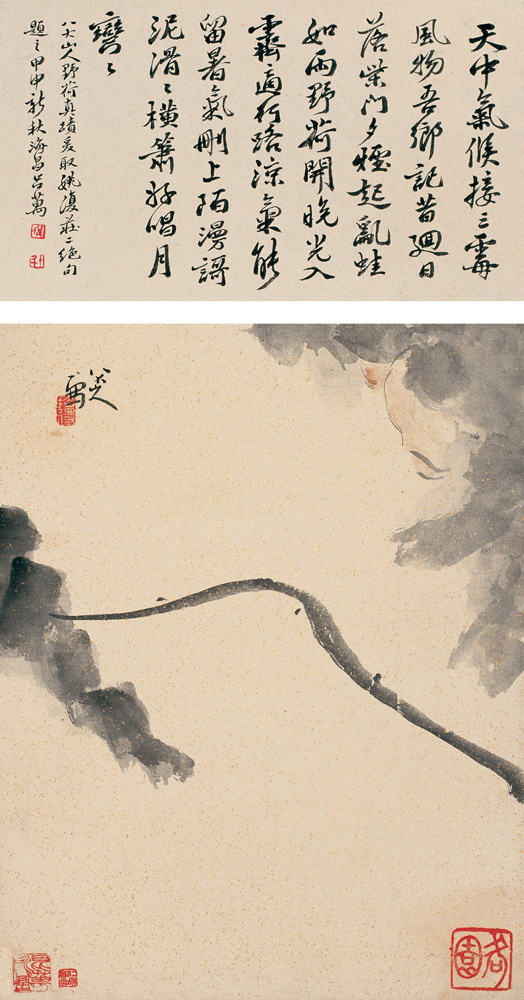The artwork is a traditional Japanese print that combines a written narrative and a richly detailed illustration. The top portion of the image is dominated by vertical Japanese characters arranged in ten rows, set against a tan or cream background. This calligraphy potentially tells a story or provides context for the visual elements below. The lower section of the print transitions into an intricate design featuring a vivid depiction of a pink sky filled with swirling gray clouds. Among these clouds, there appears to be a large, undulating shape that resembles the Great Wall of China. On the left side, a distinctive red figure with black tentacle-like appendages extends towards the right, creating an intriguing focal point. Additionally, there's an enigmatic gray string-like formation emanating from the left side and stretching diagonally downward. In the lower corners of the print, more Japanese symbols can be found—two in the left corner and one in the right corner. Intriguingly, within the cloudy formations, one can discern the face of an Asian man adorned with an elongated mustache flowing down to his chin, adding a mysterious and human element to the ethereal scene.